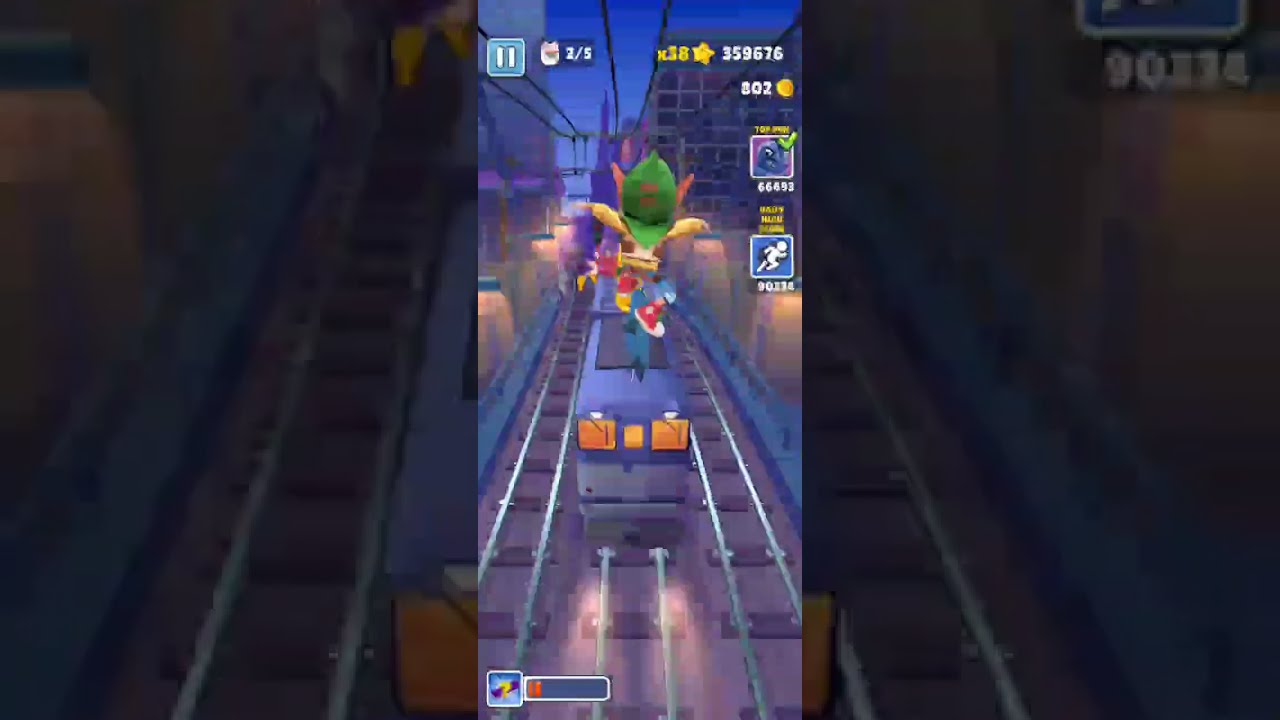The image is a detailed screenshot from a popular mobile video game, likely a screen grab from a gaming channel. The scene captures a fast-paced urban setting at night, characterized by a bluish hue. The main focus is on a character who is mid-jump onto the roof of a centrally located train, navigating a city filled with obstacles. The character, seen from behind, sports pointed ears, a green baseball cap, red shoes, and is wearing a yellow jacket. 

The train, which has orange windows and is purplish-blue in color, runs along grayish tracks surrounded by a cityscape with buildings, lit lamp posts, and electrical wires. The urban environment is detailed with multiple colors including green, red, blue, gray, orange, black, and purple.

Overlaying the scene are game interface elements: a bright turquoise blue pause button at the top left with "2 out of 5" levels indicated, followed by a star with "38" points next to it. Additional statistics display "359676" above "802" with a coin icon, and "90114" with a running man icon. There's also a red health or life stat bar at the bottom left. Together, these elements blend to create an immersive and action-packed visual of the gaming experience.